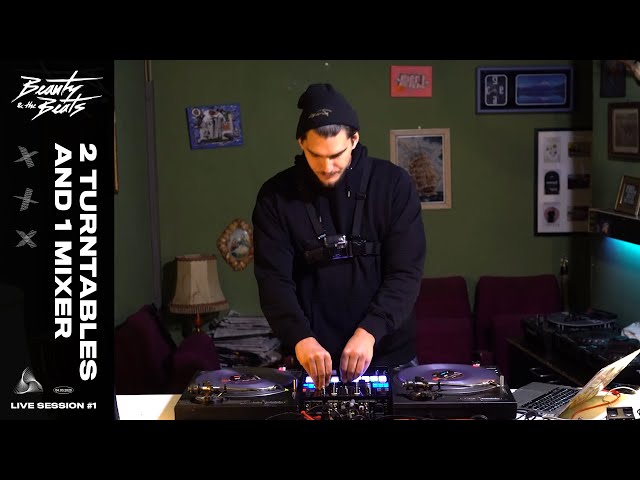In the image, a young man is deeply engrossed in operating a DJ turntable setup. This setup includes two distinct places for records on the left and right sides and an array of glowing blue and white buttons and several protruding silver knobs centrally located on the mixer. He is attired in a long black shirt, possibly overalls, and a black hoodie, with a black ski cap covering his head as he concentrates on his task. He is also seen with glasses and a strap of some sort, which might be for a camera or another accessory. His body faces the viewer, but his head is bent down towards the equipment.

The background features a dark green, almost olive-colored, wall adorned with various unique photos and posters. To the left of the man, there’s a lamp, and to the right, faintly visible, is another DJ setup on a desk. In the room, which resembles a living room or bedroom, there are dark red chairs adding a touch of color and a sense of coziness. A laptop, which the man occasionally glances at, sits on the table beside the turntables.

Overlaying the image are several texts: "Beauty and the Beats" is elegantly inscribed in cursive at the top, "two turntables and one mixer" is presented in white text on the left side, and "live session number one" is marked at the bottom, all contributing to a cohesive and organized setup for what appears to be a live DJ session. The image is framed by horizontal black stripes at the top and bottom and a vertical black stripe down the left side, adding a sleek border to the overall scene.